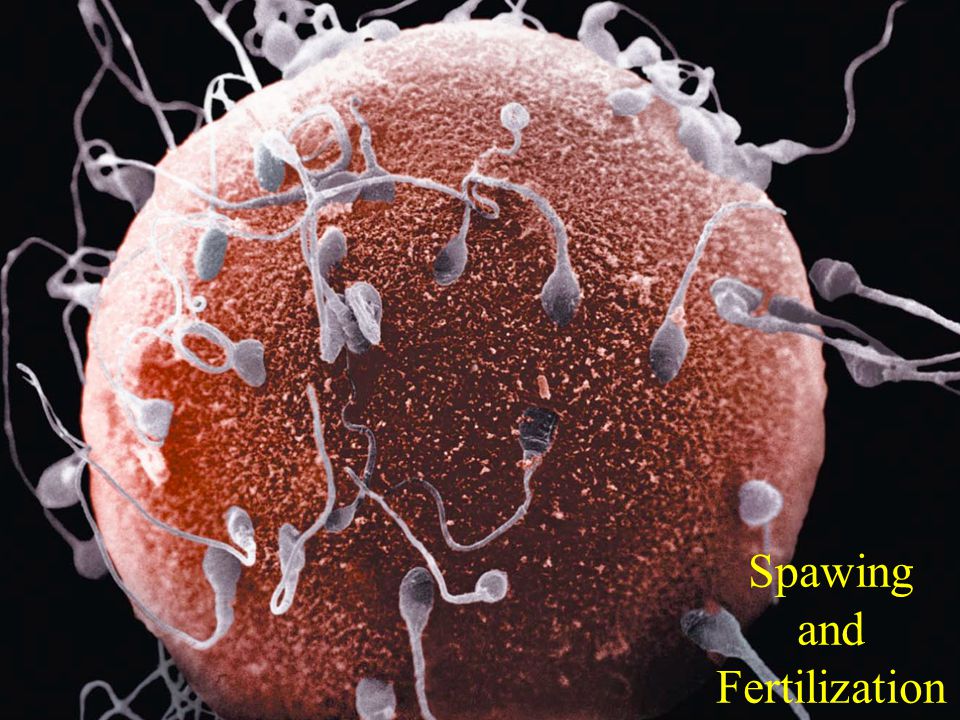The high-definition photograph captures an intricate stage of human fertilization against a solid black background, creating a stark visual contrast. Dominating the frame is a reddish-orange human egg with a rigid, rough surface, around which numerous sperm cells are converging. The sperm cells are detailed with light to dark gray heads and winding, flagella-like tails extending in various directions as they target and attach to the egg. In the lower right corner, yellow-gold text reads "Spawning and Fertilization," providing a clear caption for this striking and detailed image.